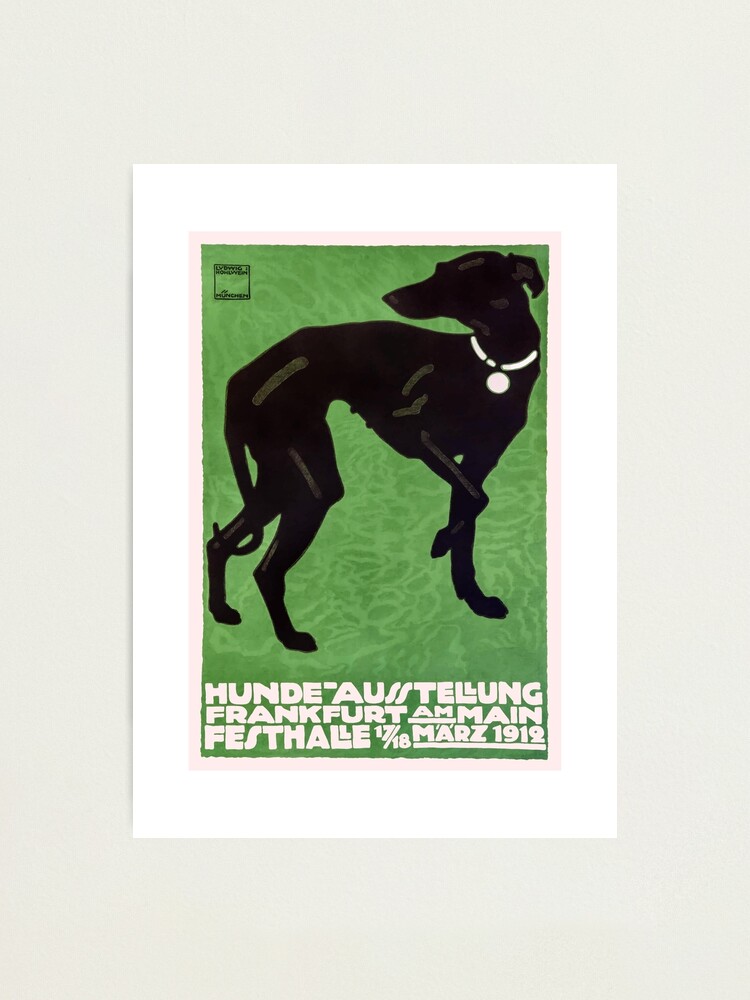The image is a vintage-style poster with a thick white border framing a central green rectangle. Within the green background is a black dog, depicted in a poised stance, looking to the left with one leg raised as if in motion. The dog wears a white collar with a circular tag hanging from it. The dog's facial details are obscure, rendering the entire figure in silhouette. In the top left corner of the green rectangle is a small black box containing some text. The bottom of the green rectangle features writing in what appears to be German, including phrases such as "Hund Achtelung Frankfurt am Main, Festtage 1718," or variations like "Honda Stahlung Frankfurt am Main Vestal 17 over 18 Mars 1912." The writing is in thick, white, capital block letters. The overall composition suggests a simple yet artistic design.